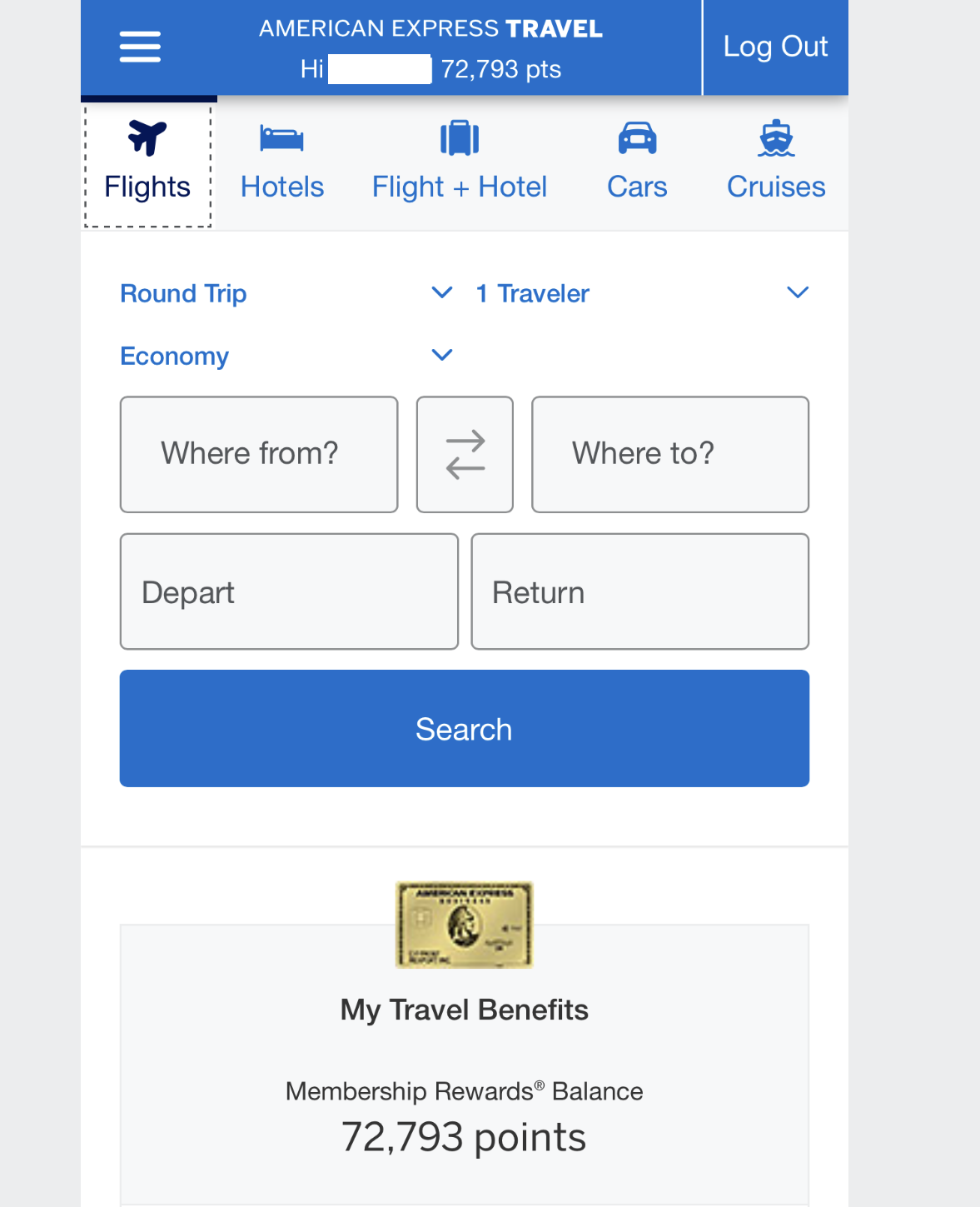Screenshot of American Express Travel App - Flight Section:

At the top of the mobile screen, a blue bar spans across the width, featuring key navigation elements. On the far left, a white hamburger menu icon (three horizontal lines) is visible. Centrally positioned is the heading "American Express TRAVEL," where "American Express" is in standard font weight, all capitalized and white, while "TRAVEL" is in bold, also capitalized and white. A vertical line separates this from the "Log Out" option on the right, displayed in white letters on the blue background.

Below the main heading, user-specific information is partially visible. The greeting "Hi," is followed by a user-edited white rectangle obscuring the name, with "72,793 points" displayed to the right of the obscured name.

The app features a horizontal navigation bar for different travel options. The current section is highlighted with a dotted square around the selection:

- An airplane icon labeled "FLIGHTS" in either black or very dark blue text on a white background (current selection).
- Other options include "HOTELS" with a bed icon, "FLIGHTS & HOTELS" with a suitcase icon, "CARS" with a car icon, and "CRUISES" with a cruise ship-front icon, all presented on a light gray background.

The main content area of the app consists of input fields and selection options for booking a flight. On the left, two dropdown menus are labeled "Round Trip" (in blue text) and "Economy." On the right, a dropdown labeled "1 Traveler" is present.

Further down, input fields for flight details appear in two rows:
- The first row has three fields: "Where From" with a black rounded rectangle outline and light gray interior, a middle field with two arrows pointing left and right, and "Where To."
- The second row includes "Depart" on the left and "Return" on the right.

Below these input fields is a prominent blue button with rounded corners, featuring the word "Search" in white letters.

At the bottom center of the screen, a small image of an American Express card in golden bronze with black details is displayed, though the details are too small to discern. Below the card, text reads "My Travel Benefits" followed by "Membership Rewards Balance: 72,793 points."